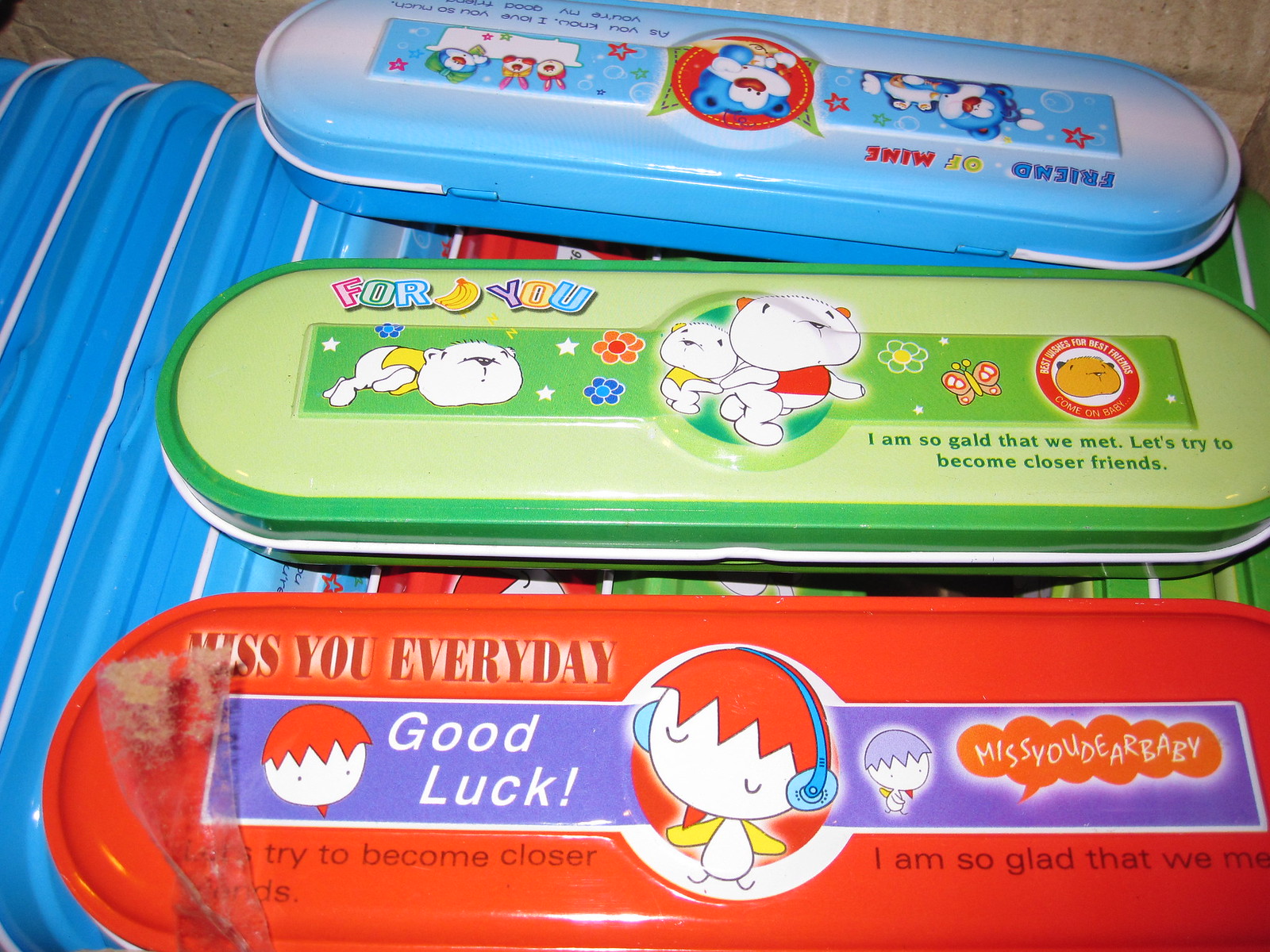The photograph captures a collection of colorful metal pencil case tins stacked horizontally inside an open cardboard box. Among these, three tins have been pulled out and placed on top of the stacks, laying horizontally. The first tin, positioned at the bottom, is predominantly red. This tin features several lines of text: "Miss you every day" in the top left corner, "Good luck" to the left featuring a boy's head with brown hair and a girl in a green sweater with headphones, and "Miss you dear baby" on the right with a smaller image of the same boy now with blue hair. 

The second tin, in the center, is green and prominently displays the words "For you" separated by cartoon bananas. It continues with a sentence at the bottom right that reads, "I am so glad that we met. Let's try to become closer friends," although "glad" is misspelled as "gald." The tin is adorned with images including a white bear with a green vest laying down, various flowers and stars, and another bear cub wearing a green vest alongside an adult bear in a red shirt.

The third tin is blue and has been placed upside down, making the text harder to read. It features the words "Friend of mine" and seems to include images of a blue cat with a red nose lying down and possibly red rabbits. Decoration includes red, green, and blue stars, along with text that partially reads "As you know, I love you so much, you're my good..." The style and elements of these tins suggest they are intended as heartfelt, perhaps nostalgic gifts, adorned with colorful imagery and messages of friendship and affection.